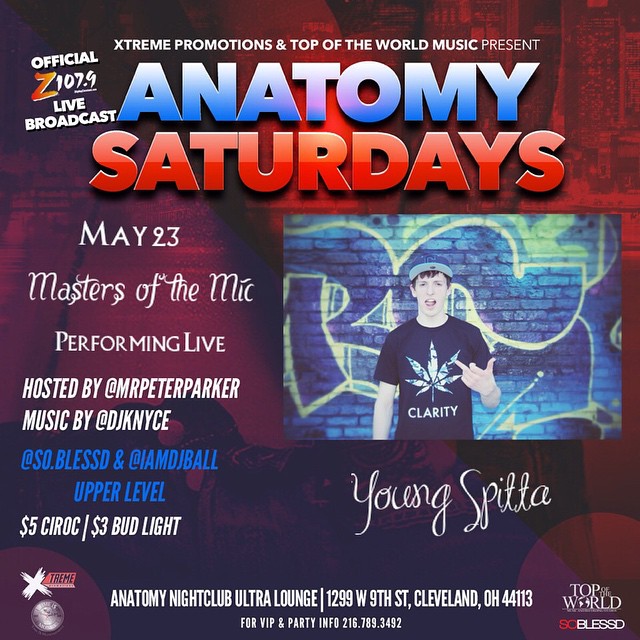The advertisement, filled with various details, promotes a live performance at Anatomy Nightclub, Ultralounge, located at 1299 West 9th Street, Cleveland, Ohio, 44113. The background of the image transitions from a red-filtered city skyline at the upper right to a darker, bluish tint toward the bottom left. At the top, bold white text announces "Extreme Promotions and Top of the World Music Present," followed by large blue letters spelling "Antenna Anatomy," with "Saturdays" in red below.

On the left side, the advertisement highlights "Official Z 107.9 Live Broadcast" in white text and mentions the event details: "May 23, Masters of the Mic Performing Live, hosted by @MrPeterParker, Music by @DJKNYCE." Further down in blue text, it lists "@SoBlessed & @IAMDJBall Upper Level." The promotional offers include "$5 Ciroc" and "$3 Bud Light."

On the right side, there is a photograph of a man standing against a graffitied brick wall. He is wearing a beanie with a green bottom and white top, a black shirt emblazoned with a marijuana leaf, and the word "Clarity" underneath. The man, with an open mouth and tongue sticking out, is holding up his left hand with the middle finger extended in an obscene gesture. Below the photograph, the name "Yalvzy Spitta" appears in flowing cursive text.

At the bottom, practical information in white text includes "Anatomy Nightclub, Ultralounge, 1299 West 9th Street, Cleveland, Ohio, 44113. For VIP and party info, call 216-789-3492." The image is embellished with logos and additional text: the "Top of the World, BC Blessed" logo in the bottom right corner, and an "X Dream" graphic with a silver coin on the bottom left. The extreme promotions logo and a small patterned circle are also featured.